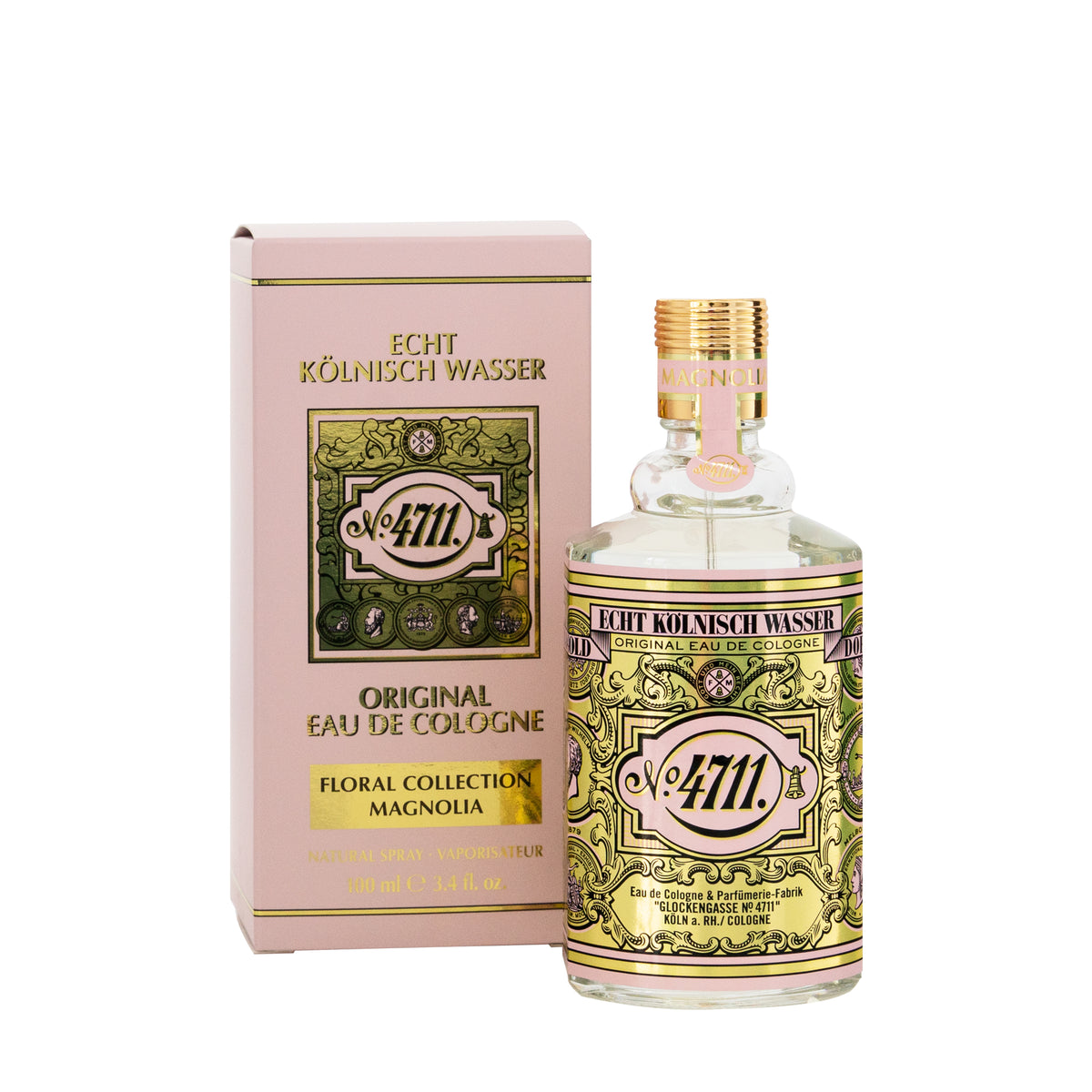This detailed photograph showcases a crisp and clear image of a bottle of Cologne along with its packaging. The light pink box, adorned with gold lettering and an intricately ornate pattern, is positioned on the left side of the image. It prominently features the phrases "Echt Kolnisch Wasser," "4711," and "Original Eau de Cologne Floral Collection Magnolia." Most of the text is in German, with some parts not entirely legible, except for an address including the word "Glockengasse." On the right side, the clear bottle mirrors the box’s aesthetic, flaunting a matching pale pink and gold label intricately decorated. The bottle’s label reiterates the branding with "4711" and "Echt Kolnisch Wasser" alongside similar florals and patterns. Its gold cap, topped with what appears to be a tamper-proof seal, completes the elegant design.